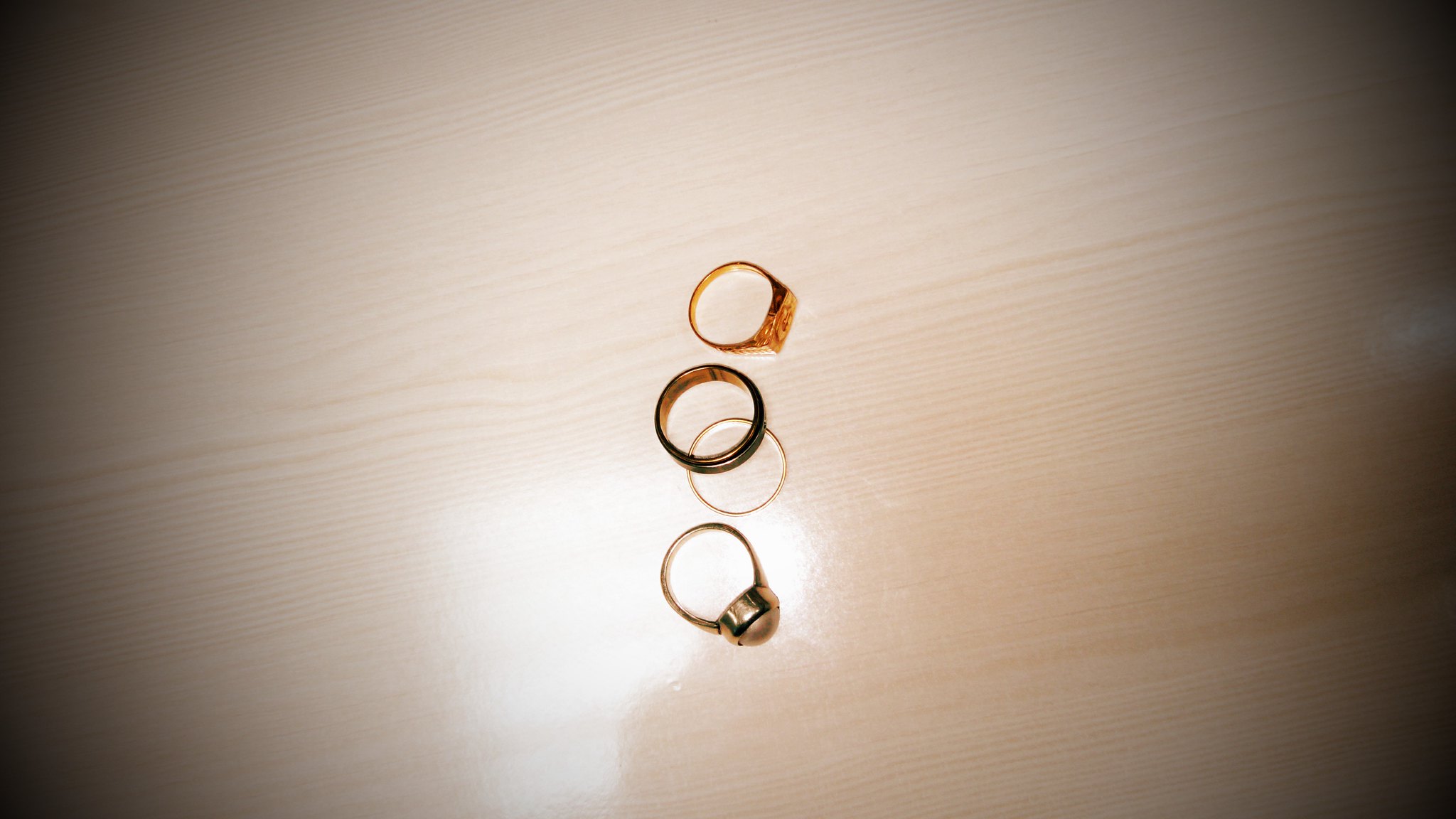This is a detailed photograph taken from above, showcasing a polished, ashen white wooden tabletop that has a distinct silver or shiny appearance, possibly resembling wood grain or wrinkles in a cloth in the background. The image is in landscape mode with black shadowing in the top left, top right, bottom left, and bottom right corners, creating a vignette effect around the edges. 

In the center of the table, four rings are neatly displayed in a vertical arrangement. At the top, there is a gold ring with a flat, square medallion setting. Below it, a black band ring with a gold interior is positioned. Underneath the black ring, there is a very thin gold ring. At the bottom of the arrangement, a shinier, brass-colored ring with a round, dark rose-colored gem or globe-like setting is featured. The careful arrangement and detailed lighting bring out the characteristics and textures of each ring, emphasizing their unique designs against the subdued yet elegant background.